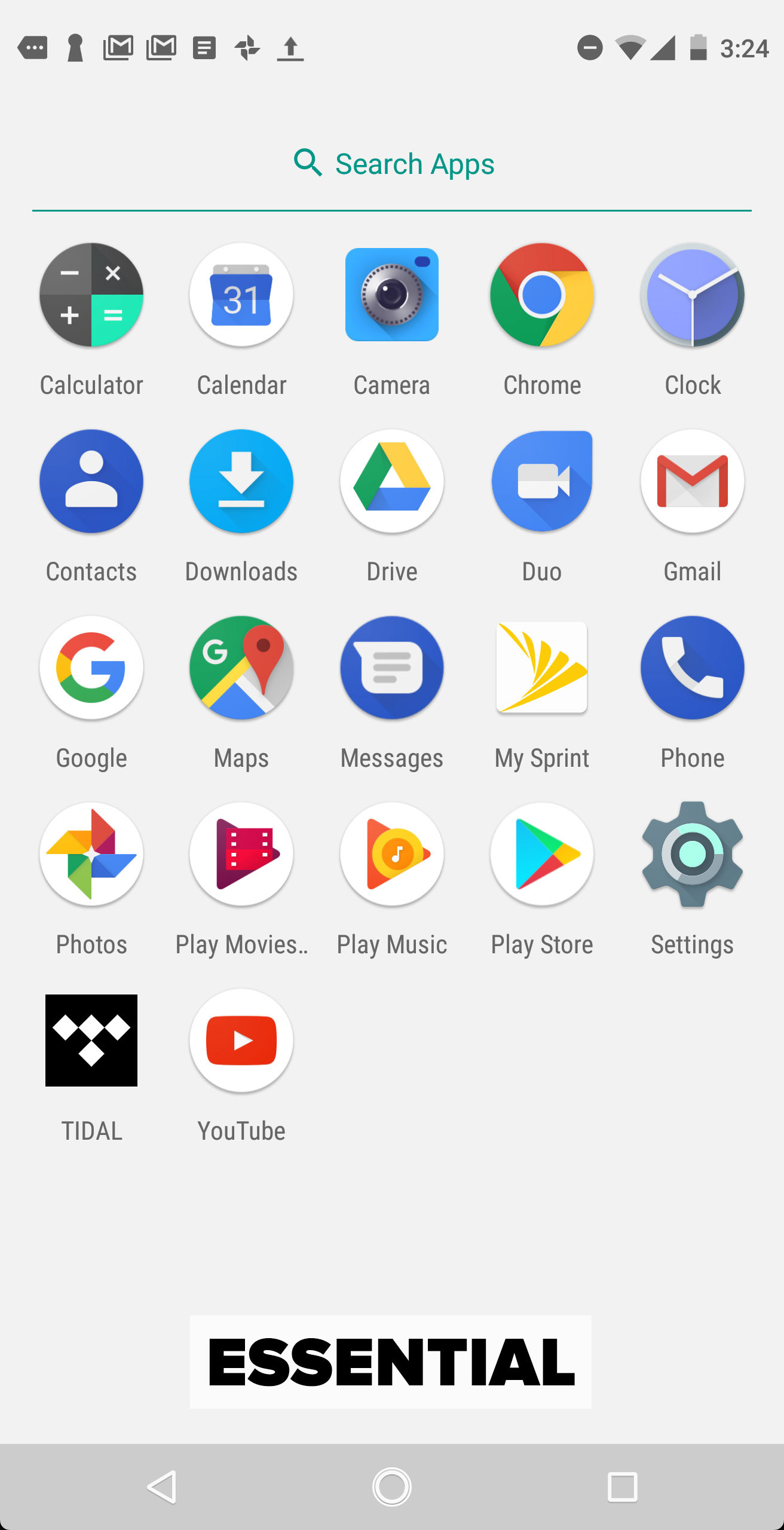The image showcases a typical Android home screen featuring a well-organized grid of app icons for effortless access. At the top of the screen, a search bar facilitates quick app searches. The app icons are neatly arranged in rows to maximize functionality:

- **Top Row:** Calculator, Calendar, Camera, Chrome, Clock
- **Second Row:** Contacts, Downloads, Google Drive, Google Duo, Gmail
- **Third Row:** Google, Google Maps, Messages, My Sprint, Phone
- **Fourth Row:** Google Photos, Play Movies, Play Music, Play Store, Settings
- **Bottom Row:** Title, YouTube

Below the app icons, a multi-functional navigation bar includes the essential controls - a triangle, a circle, and a square for seamless home screen navigation.

At the very top of the screen, the system tray displays pertinent information such as the current time (3:24), battery level, signal strength, and Wi-Fi connectivity. 

Positioned at the bottom of the screen, there appears to be branding that possibly identifies the device model or manufacturer, referred to as "essential" in the image.

Overall, this interface provides a clean, organized layout that enables users to access frequently used apps quickly, offering an intuitive experience by reducing the need to scroll through multiple screens.